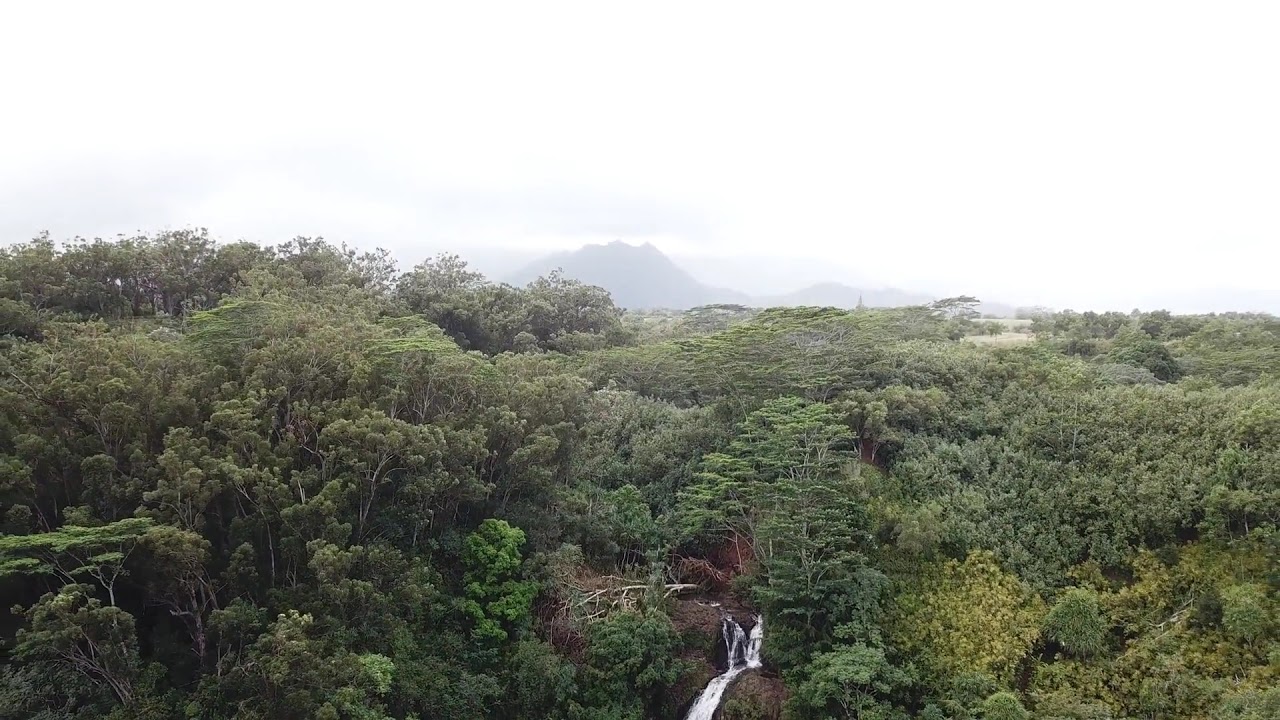The image captures an expansive aerial view of a dense, lush forest that could be part of a rainforest, reminiscent of scenes from "The Lion King" with its distinct shelf-like trees. The forest canopy is a rich tapestry of dark green, light green, and yellow foliage. Towards the bottom center of the image, there is a charming, small waterfall, its presence creating a focal point in the verdant landscape. Beyond the tree line, high hills or mountains rise, partially shrouded in fog, adding a mystical quality to the horizon. The bright, white sky, dotted with a few clouds, contrasts with the dense greenery below, highlighting the vertical expanse. On the left side, the forest appears particularly dense, with trees vying for space, while the right side transitions to bushier scrubland. A pathway is visible at the forefront, bordered by patches of cleared, empty dirt, suggesting human activity.